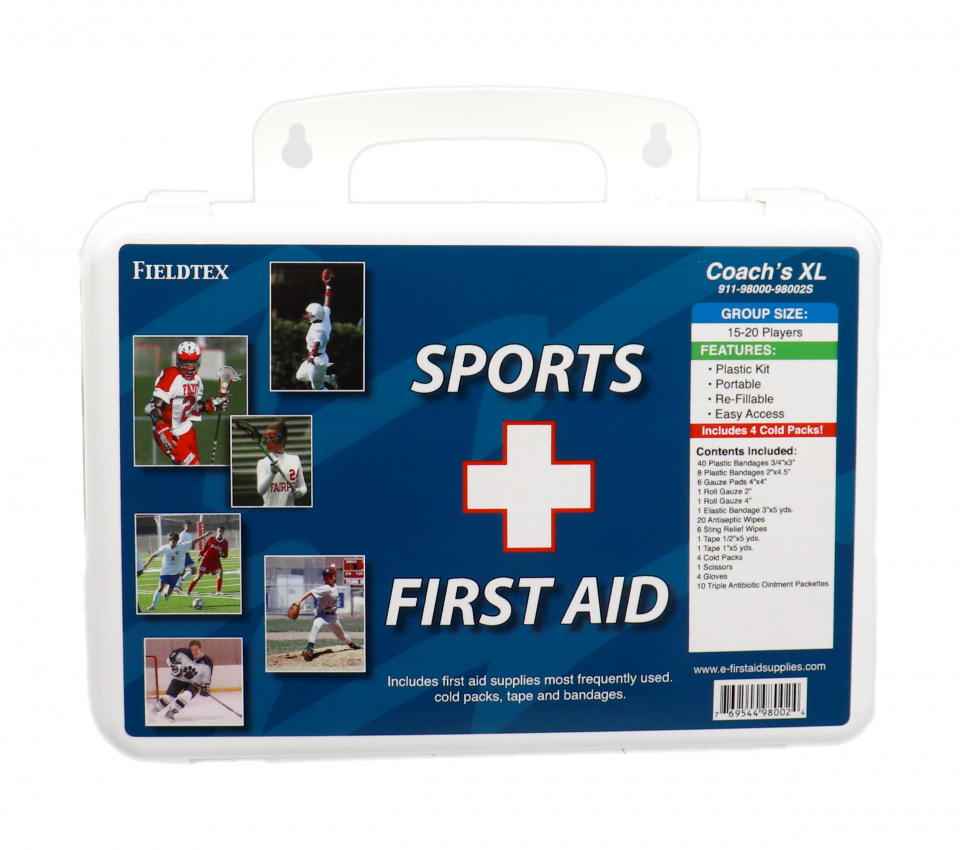The image depicts a first aid kit designed specifically for sports teams, branded by Fieldtex. The kit itself is white with a large blue label across the front, featuring the words "Sports First Aid" prominently displayed alongside a white cross outlined in red, signaling first aid. It is labeled as "Coach's XL," intended for coaches, and is suitable for groups of 15 to 20 players. The label details that the kit includes frequently used sports first aid supplies such as cold packs, tape, and bandages. It is designed to be portable, refillable, and easy to access, contained within a durable plastic case. In the upper left corner, the Fieldtex logo is present, just above a series of six images depicting young male athletes participating in various sports including football, lacrosse, soccer, baseball, and hockey. A barcode and a partially legible website are located on the bottom right-hand corner of the label. The left side of the label displays what appears to be photos resembling playing cards, depicting the youth athletes in action, emphasizing the versatile applicability of the kit in different sports settings.